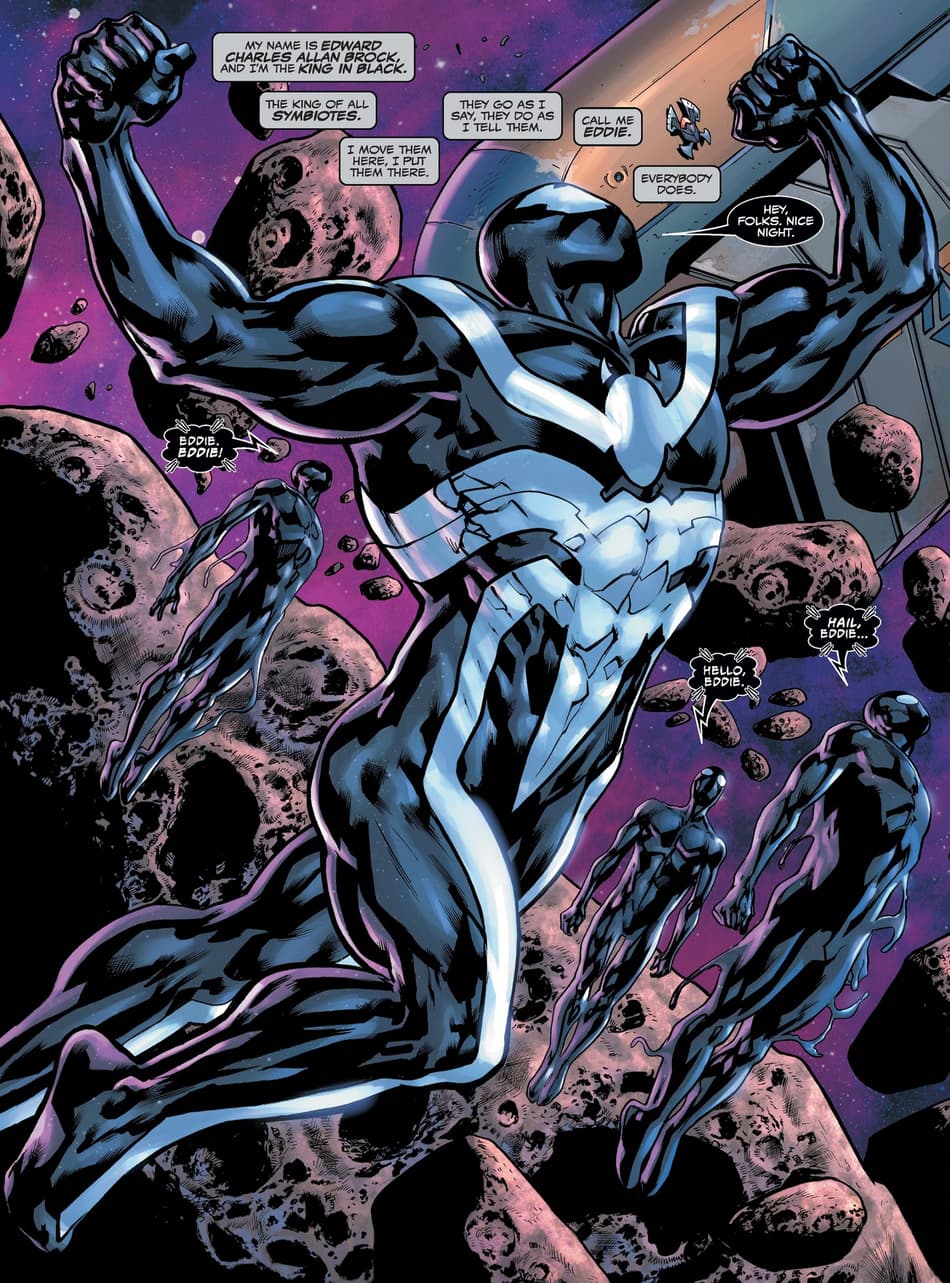The image is a rectangular comic book page, approximately 6 inches high and 4 inches wide, and features a vividly illustrated scene in a cartoon-like style. The central character, seemingly Venom, dominates the composition. He is dressed in an extremely tight black latex-like bodysuit adorned with a large white spider emblem, its legs extending over his shoulders and down his chest and legs. His attire is so form-fitting that it accentuates his powerful, muscular physique, making it appear as though he is almost naked, his skin painted with symbolic patterns. His face is masked, revealing large spider-like eyes, giving him a menacing, bug-like appearance. 

This main figure is identified through speech bubbles scattered across the sky-like background, a blend of purple and gray hues stretching diagonally, accompanied by floating brown asteroids. The character introduces himself as "Edward Charles Allen Brock, the king in black, the king of all symbiotes," asserting his control over the symbiotes with lines like, "I move them here, I put them there. They go as I say, they do as I tell them. Call me Eddie. Everybody does." He cheerfully adds, "Hey folks, nice night," in a larger speech bubble.

Surrounding Eddie are similar figures, seemingly symbiotes or symbiote-influenced beings, clad in black bodysuits with possible variations in color patterns, such as black and gold or black and silver, and possessing minimal facial features aside from large, smoothed-over eye segments. These figures float in the space-like environment with their arms by their sides, forming a dynamic yet somewhat eerie assembly. They echo Eddie's name in unison through their speech bubbles with phrases like, "Eddie, Eddie, hello Eddie, hail Eddie," underscoring his dominance and their collective identity.